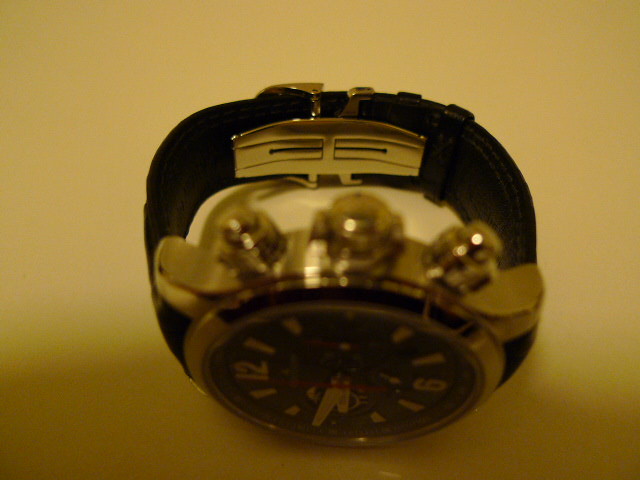This close-up, horizontally oriented photograph captures a chronograph-style wristwatch against a yellowish, possibly tinted background. The watch features a dark-colored face with white numerals, prominently displaying the time at approximately 9:45. Three dials are visible on the left side of the watch—two push-buttons and a central rotatable knob—for adjustments, though slightly out of focus. The watch body appears to be a metallic silver or gold, influenced by the lighting, and is framed by an aluminum or chrome bezel. The thick rectangular hour and minute hands are white. The watch's black leather band is secured with shiny metallic, gold-accented clasps.